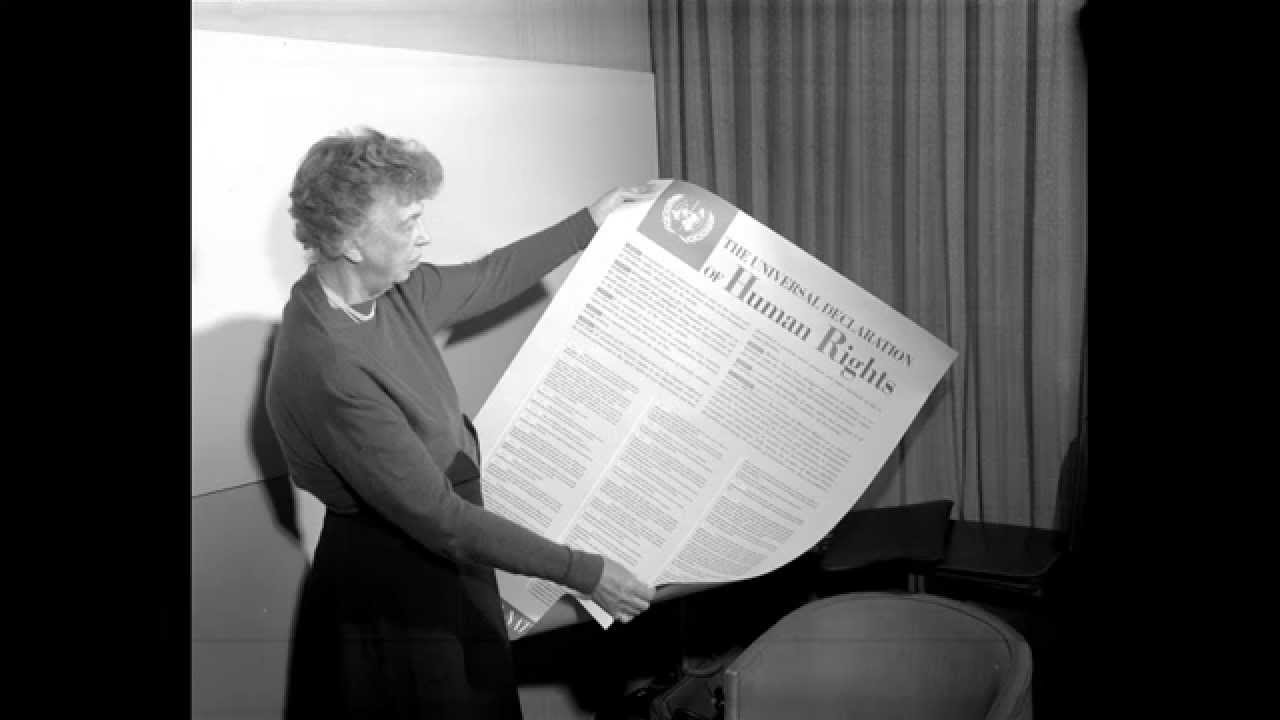The black and white photograph features Eleanor Roosevelt, an older woman with short, curly light brown hair, standing in a room with white walls and draperies hanging up. She is dressed in a long-sleeve dark sweater and a dark skirt, accessorized with a string of pearls around her neck. Eleanor is prominently holding a large poster, nearly the size of her body, displaying the title "The Universal Declaration of Human Rights" at the top, with the United Nations logo to the left of the title. The poster contains extensive small print, indicating the detailed content of the declaration, underscoring her significant role in presenting and advocating for this historic document at the United Nations.